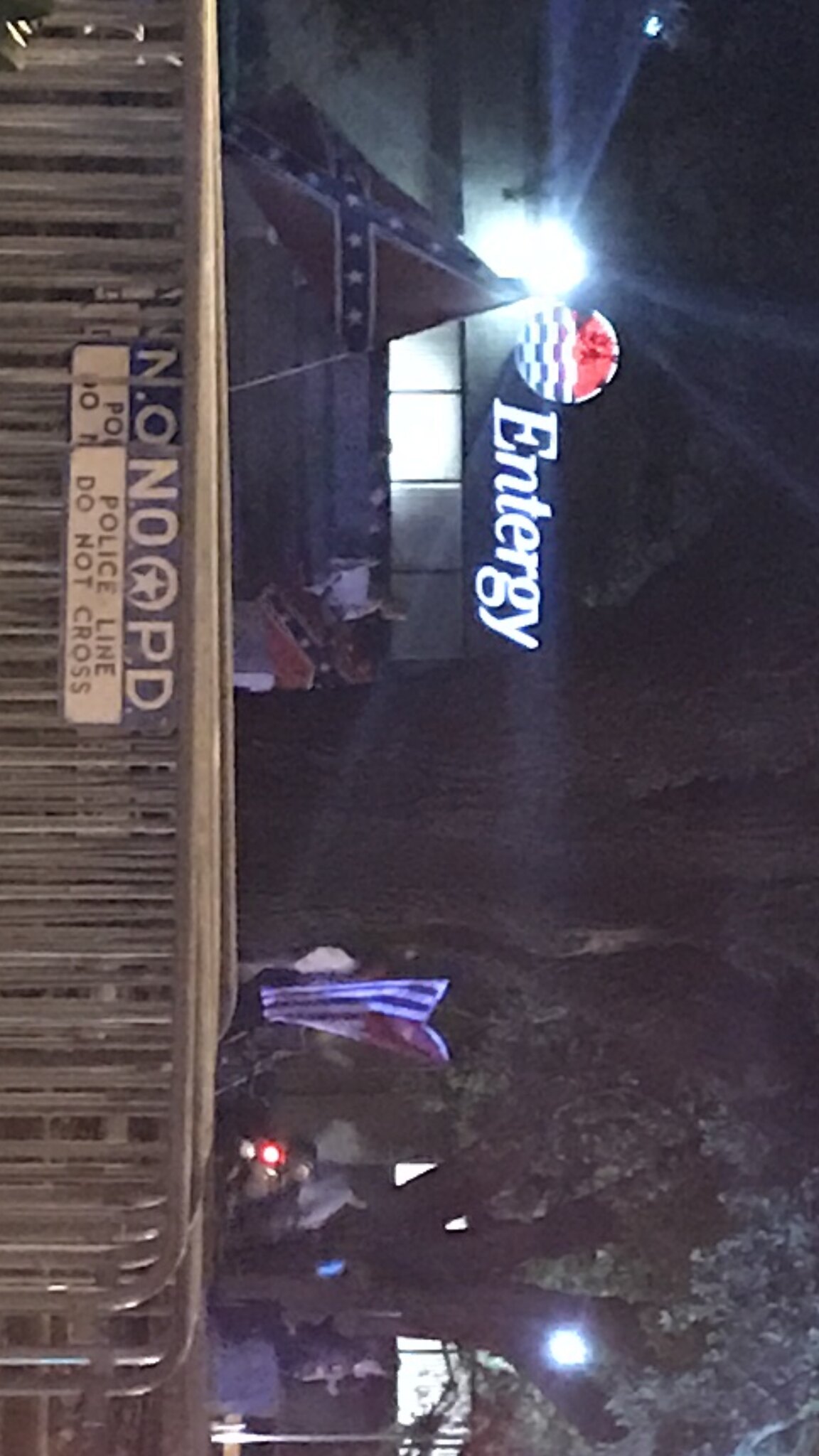This photo, taken outdoors and rotated 90 degrees to the right, captures a scene in front of a building marked "Entergy." A man stands at a podium draped with a Confederate flag. A flagpole nearby also displays a Confederate flag. Metal barrier gates are stacked in the background, featuring signs that read "No PD Police Line Do Not Cross." The environment includes large trees, and the Entergy building is notable for its distinctive design, featuring a red circular element at the top and black and white striped patterns beneath silver windows.